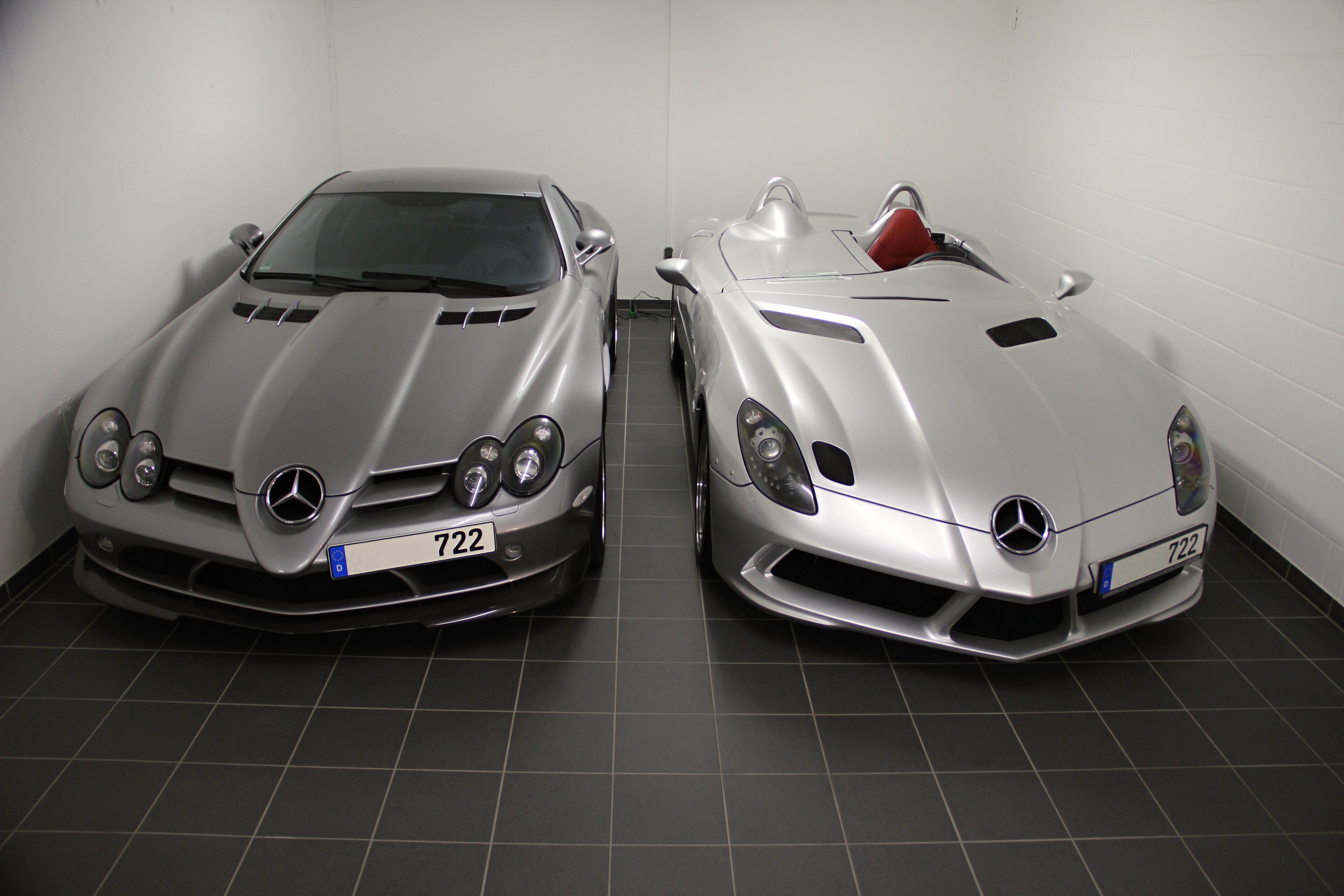The room features stark white walls with subtle grey accents and a sleek black tiled floor. Inside, two silver vehicles are on display, each with distinctive characteristics. The vehicle on the left is a darker shade of silver and is outfitted with a white license plate bearing the number "722" in black text. It boasts four headlights and tinted windows. The vehicle on the right, lighter in silver, shares the same "722" license plate but stands out with only two headlights and a single red seat visible from outside. Both vehicles display circular emblems divided into three sections at the front.